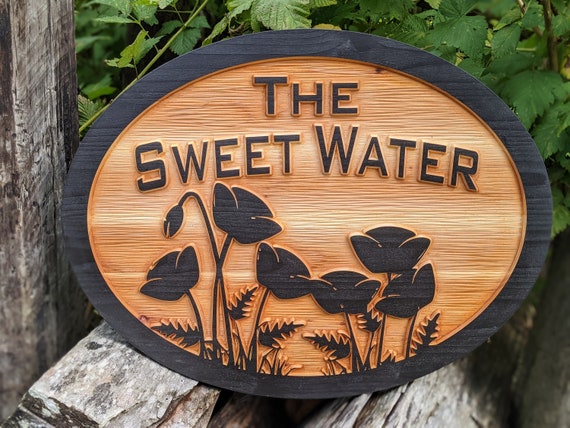The image depicts a close-up of an oval-shaped, wooden sign with a noticeable wood grain and a smooth, black-painted border. The natural wood color fills the background inside the border. The sign, which appears to be machine-carved rather than hand-carved, displays the text "The Sweetwater" in black paint over a roughly textured, etched surface. Beneath the text, there are black-etched or embossed images of seven flowers, complete with stems and leaves. The sign rests on two pieces of stacked, light-colored wood, resembling logs or firewood. Surrounding the sign, the background is filled with dense, dark green foliage, and a grayish pole is visible to the left. There is no additional text indicating what establishment the sign represents.